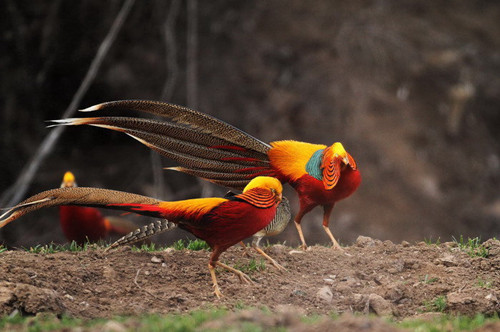In this photograph taken during the daytime, three distinct birds stand on a ground full of brown dirt. Two prominent golden birds with elongated brown tails and yellow heads face to the right. The bird in the front displays a striking red wing, while the bird in the back turns its head slightly, revealing a hint of blue near its top and two slender necks. Between these two, a smaller grey bird is visible. The vibrant birds, adorned with shades of orange, red, yellow, and green, contrast starkly against the dark, dirt-laden ground, creating a vivid and captivating scene. The tall feathers of their tails, the beautiful markings on their bodies, and their unique posing add to the image’s allure.